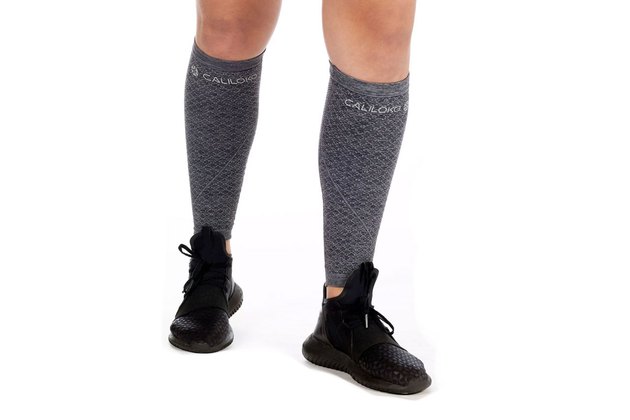The image depicts a person's light-skinned legs, shown from just above the knees to the feet, set against a transparent white background. Both legs are adorned with gray calf sleeves or compression socks that extend from just below the knees to around the ankles, featuring a quilted pattern. The calf sleeves bear the brand name "CaliLong" in white text at the top, accompanied by a small circular logo. The individual is also wearing black athletic shoes with high tongues and wide soles. There is an observable gap between the end of the calf sleeves and the start of the shoes, revealing a small portion of the skin above the ankles. The overall composition suggests a promotional image, highlighting both the compression socks and the athletic footwear.